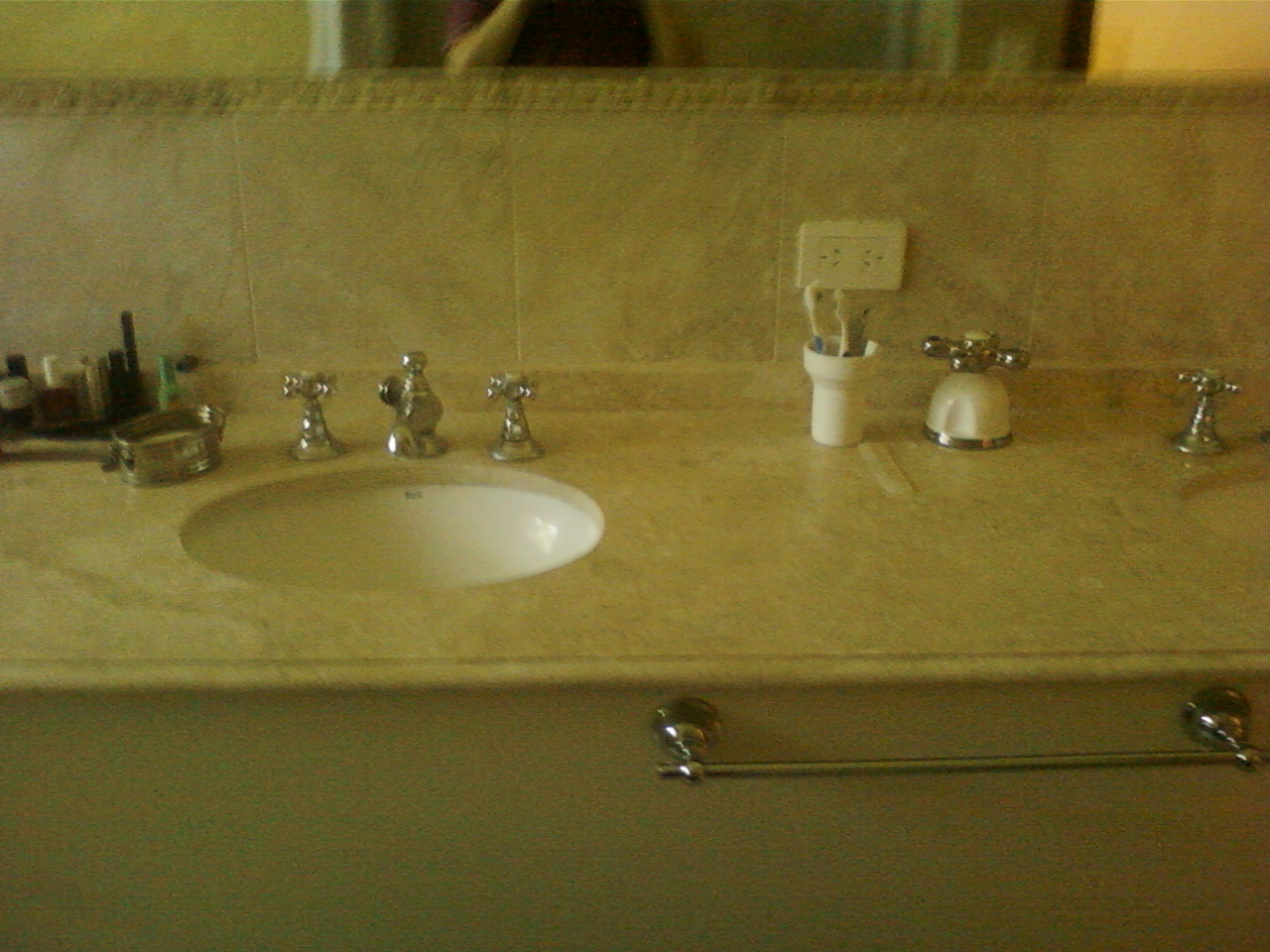This detailed photograph captures a glimpse inside a bathroom. The interior features off-white, marbled tiles that cover the lower half of the walls, transitioning to an almost yellowish off-white color above. A mirror hangs on the upper portion of the wall, though only the bottom part is visible. Reflected in the mirror is a partial image of a person, likely Caucasian, clad in a red t-shirt which reveals their chest and forearms.

The bathroom counter holds two white, round sinks with sleek silver fixtures. The left sink is fully visible, whereas only part of the right sink can be seen. Positioned between them is a white cup holding toothbrushes. Just behind the cup, there's a visible electrical outlet on the wall. Further to the left, a soap dish made of silver holds a piece of white soap. In front of the sink, a silver towel rack is mounted.

On the far left side of the counter, there is a tray brimming with various products, including an assortment of makeup items and nail polish bottles. The scene paints a thorough picture of a lived-in, functional, and organized bathroom space.